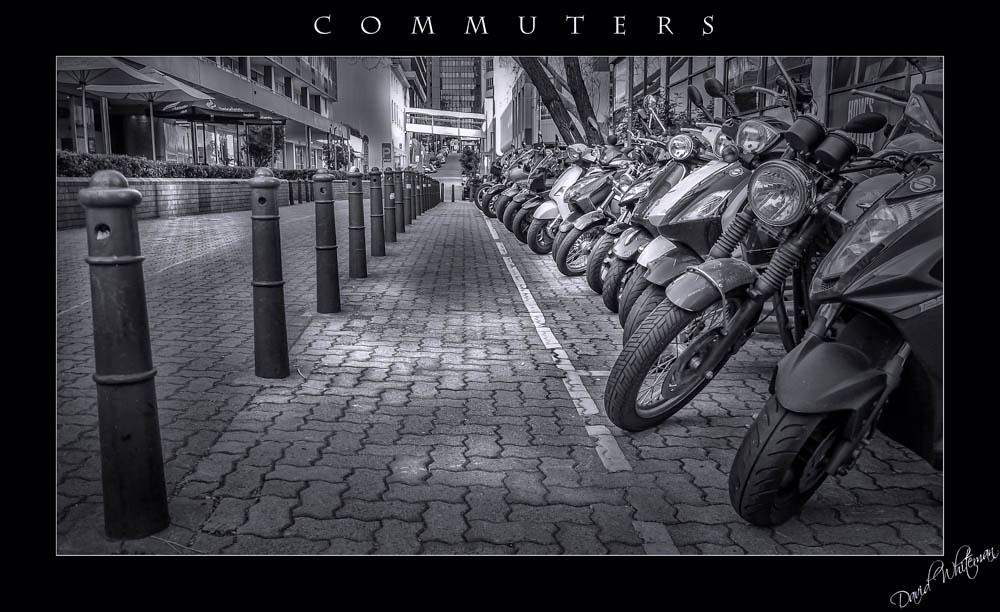A detailed black and white image captures a busy downtown area, showcasing a realistic yet artistic scene. The grayscale photo features a long, cobblestone-style sidewalk composed of intricately fitting flat stones with wavy edges. Along the left side of the sidewalk stands a series of rounded black pillars with holes near the top. To the right, a line of approximately 25 motorbikes—including motorcycles, mopeds, and scooters—are neatly parked, all facing inward with their kickstands down. Above the scene, the title "commuters" is spelled out in spaced, thin white letters. In the background, multiple-story buildings with more pillars are visible, suggesting a bustling urban environment. Additional details include parked cars, some trees, and looming skyscrapers, capturing the essence of a lively cityscape. A small artist's signature is visible in the bottom right corner, adding a final touch of authenticity to the image.